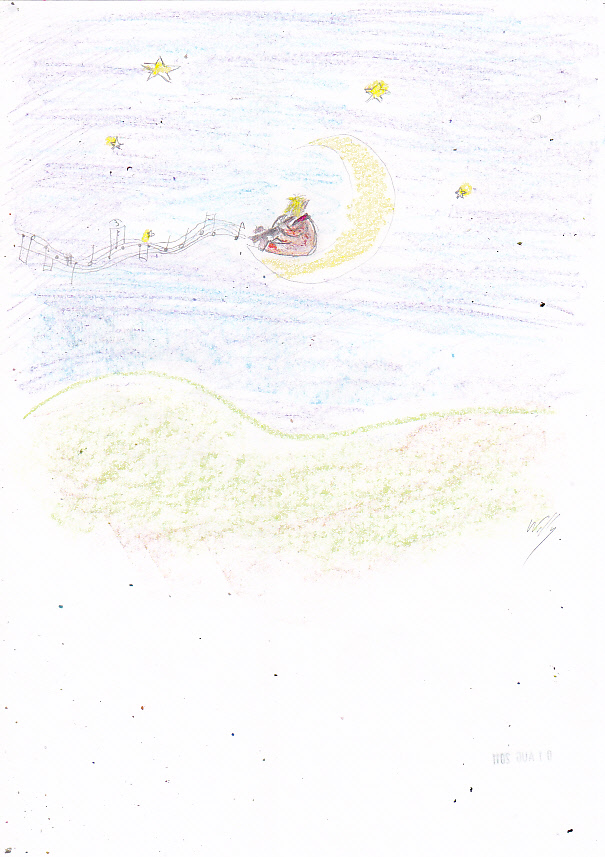This colored pencil drawing features a dreamlike scene distinguished by various vibrant hues and intricate detailing. At the bottom, a gold, wavy area forms the base of the composition. Above this foundation is a faint, soft blue section, which transitions gently into a purple center. Scattered throughout this area are shimmering gold stars that add a touch of magic to the image. Dominating the central portion is a gold crescent moon, upon which sits a humanoid figure with a golden head, adorned in a vibrant red outfit. Radiating from this enchanting character are wavy musical notes, seemingly emanating harmonious melodies. Despite the rich detail, the white background paper subtly peeks through in certain parts, adding depth to the artwork. The lower part of the drawing includes an artist's signature, although it is quite small and partially obscured, making it difficult to decipher.